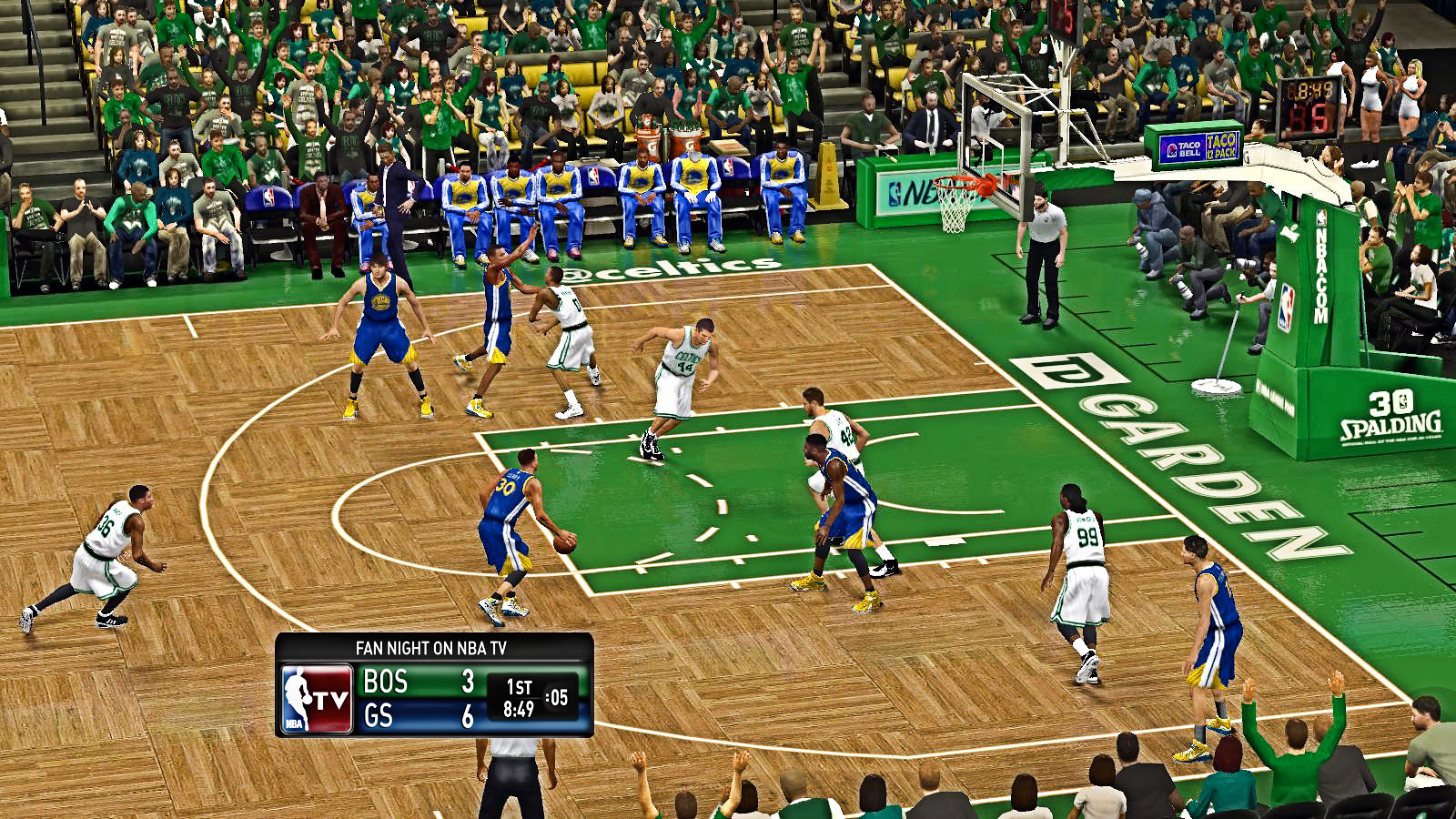The screenshot captures an intense moment of a basketball game in progress at TD Garden, identifiable by the "TD Garden" text prominently displayed. The court's rich brown wood floor is accented with green decorations, indicative of a home game for the Boston Celtics. The two competing teams are distinguishable by their uniforms: one team in blue and yellow, and the other in white with green lettering. The vibrant atmosphere is emphasized by the packed bleachers, filled with fans, many donned in green, and the array of advertisements around the hoop, including "3D Spaulding" and "NBA.com." To the right side of the court, a coach stands, and a row of blue and gold-uniformed players await their turn. The scoreboard, located in the lower left-hand corner, displays a score of 'BOS 3' and 'GS 6,' with 0:05 left in the period and 8:49 remaining on the game clock. The arena is further highlighted with "Fan Night on NBA TV," adding to the broadcast excitement.